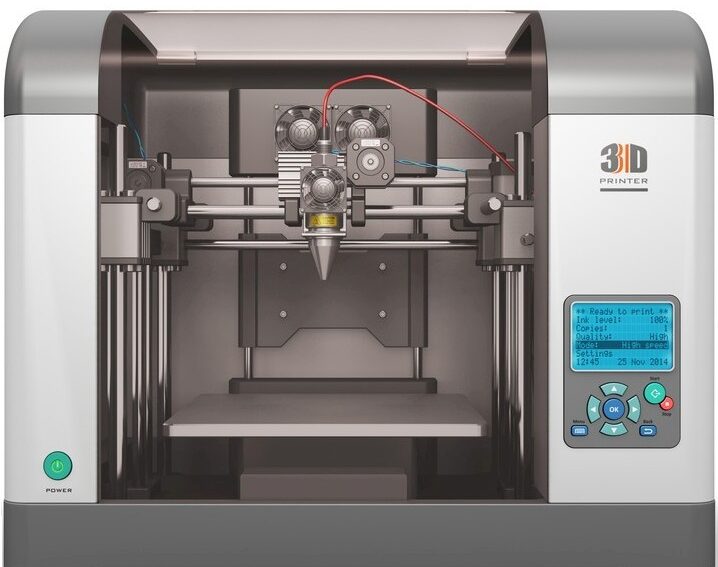The photo depicts a dissected 3D printer set against a white background, showcasing its internal mechanisms. The machine is primarily metallic silver on the top portion and gray at the bottom. On the top right corner of the printer, the label “3D” with a reddish design between the 3 and the D, followed by the word "printer," is visible on a light gray panel. The central section of the printer is open, revealing an interior crisscrossed by vertical and horizontal silver cylindrical tubes. This intricate arrangement includes a red, thin tubing leading from the right side down to a central conical nozzle. Below this machinery, we find a control panel. The control panel features a small screen with directional buttons (up, down, left, right) and a blue button labeled "OK" on the right side. Additionally, there are several other round buttons and a green power button located on the lower left-hand corner labeled “power.” Overall, the detailed internal view of the printer highlights various gears, motors, and connection points, illustrating a sophisticated and evocative look into the printer's functional components.